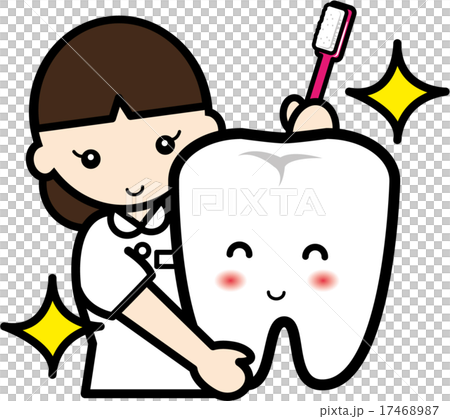The image is a cartoon drawing featuring a stylized girl on the left side, holding an oversized, anthropomorphic tooth. The girl, who has shoulder-length, even-cut brown hair with bangs, is smiling slightly. She is dressed in what resembles a white dental smock or doctor's uniform with a large semi-circle collar. In her right hand, she holds an unusually large tooth, which has a pair of arch-like eyes, a smile, and red blushing cheeks, giving it a cheerful, personified appearance. Her left hand holds a standard red toothbrush positioned over the top of the tooth. 

The background consists of a small, white and grey checkerboard pattern. Additionally, there are two yellow, four-point stars with thick black outlines: one in the upper right corner and one in the lower left corner of the image. The detail of the tooth also includes a light gray outline text that reads "PIXTA" across what appears to be the darker shaded interior of the molar, further enhancing the whimsical feel of the scene.